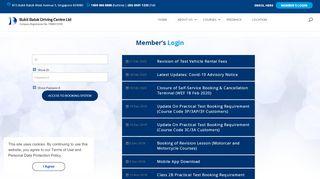The image depicts a webpage with a predominantly blue theme. At the top of the page, there's a blue header stretching horizontally across the width of the site. Within this header, there's a lighter blue box likely designed to be clickable, and it contains a search bar along with the company's name, which is unfortunately too small to decipher. The only legible text in the header is "Member's Login," positioned centrally.

Below the header, there are approximately eight dark blue bars, each containing white text. On the left side of the webpage, there are several white boxes designated for user input, where visitors are probably expected to enter information. Beneath these input fields is a blue bar with rounded edges.

The main content area of the website features various images. These images are ambiguous; they could be of people or possibly just abstract patterns formed by different shades of colors. In the bottom left corner of the page, there is a white box with black text and a clickable white circle that contains blue writing, though this text is too small to read. 

Overall, the website combines different shades of blue and white, with a mixture of text, input fields, and images, creating a visually structured, yet slightly unreadable interface.